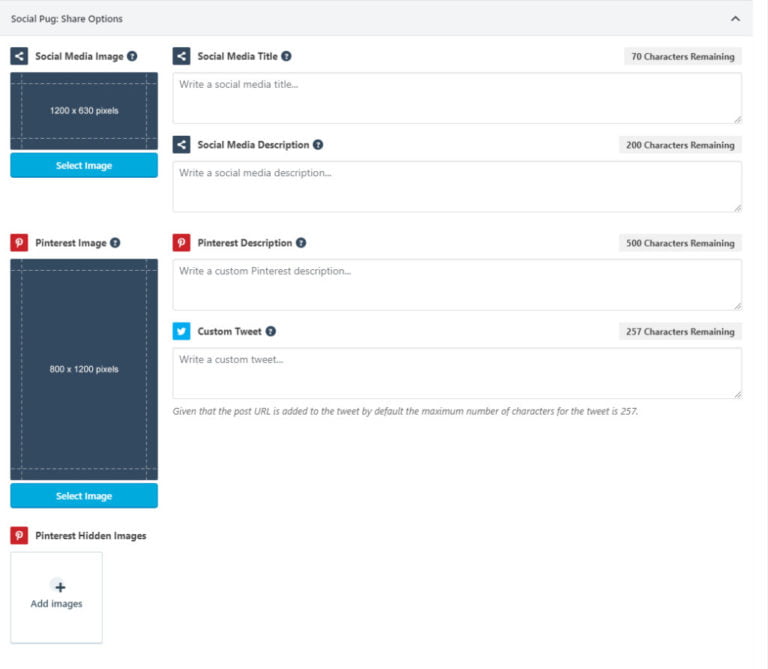A colorful landscape screenshot of a laptop or desktop computer screen displaying a Pinterest interface is shown. The screen features a form for social media image sharing options within a tool or plugin, identified as "Social Pug Share Options." The form is straightforward and functional in design, lacking extravagant aesthetics.

In the top left corner, the form is labeled "Social Media Image," with specified dimensions of 1200 by 630 pixels. Beneath this, a light blue button allows users to select an image to upload into this section. Adjacent to this, another section labeled "Pinterest Image" specifies dimensions of 800 by 1200 pixels with a similar image selection button.

Below these sections, there is an option to add hidden Pinterest images. To the right side of the form, users can input details for social media posts. The fields include "Social Media Title" with a character limit of 70, "Social Media Description" with a character limit of 200, "Pinterest Description" allowing up to 500 characters, and finally, "Custom Tweet" with a character limit of 257. Each field specifies the remaining characters as users type.